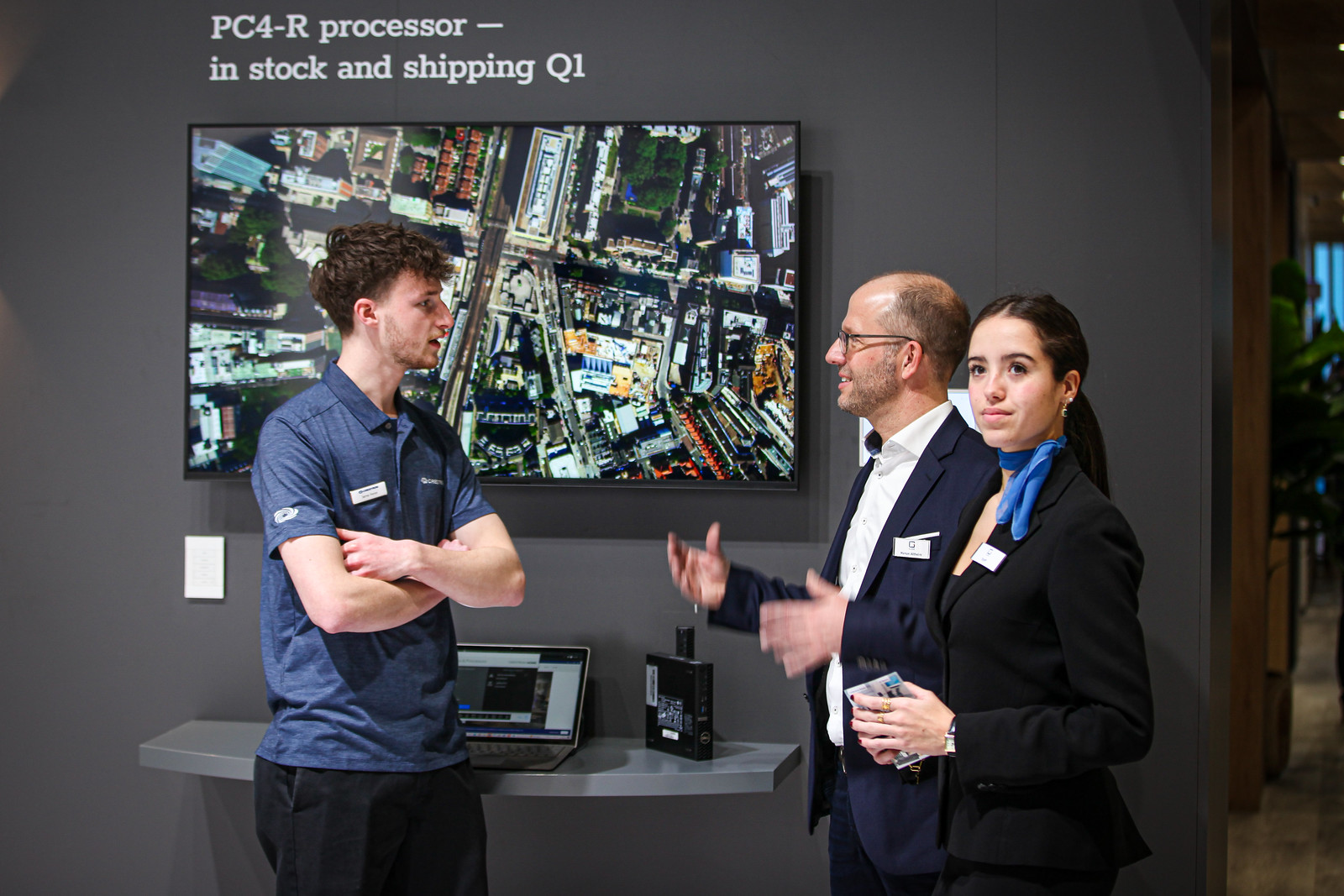This image depicts a scene at a business convention focused on technology. Central in the image, three individuals are engaging in conversation. On the left stands a young man in a corporate blue polo shirt with a logo on the sleeve and a name tag on his chest. He is wearing black pants and has his arms crossed. He engages with a man to his right, who is balding, wears glasses, and sports a light beard. This man is dressed in a suit jacket over a white button-down shirt, sans tie, and also has a name tag on his front pocket. He appears animated, gesturing with his hands.

To the right, a young woman with long brunette hair tied back in a ponytail is attentively holding a pamphlet. She is dressed in a black pantsuit, complemented by a blue scarf around her neck, and has a name tag on the lapel of her jacket.

Behind the trio, a gray wall features a mounted monitor displaying a clear aerial view of a city. Above the monitor, in white text, it reads "PC4-R Processor - In Stock and Shipping Q1." Below the monitor, a small gray shelf holds an open laptop next to a black electronic device, possibly a mini-computer. The detailed setup underscores the business and technology-focused environment depicted in the image.